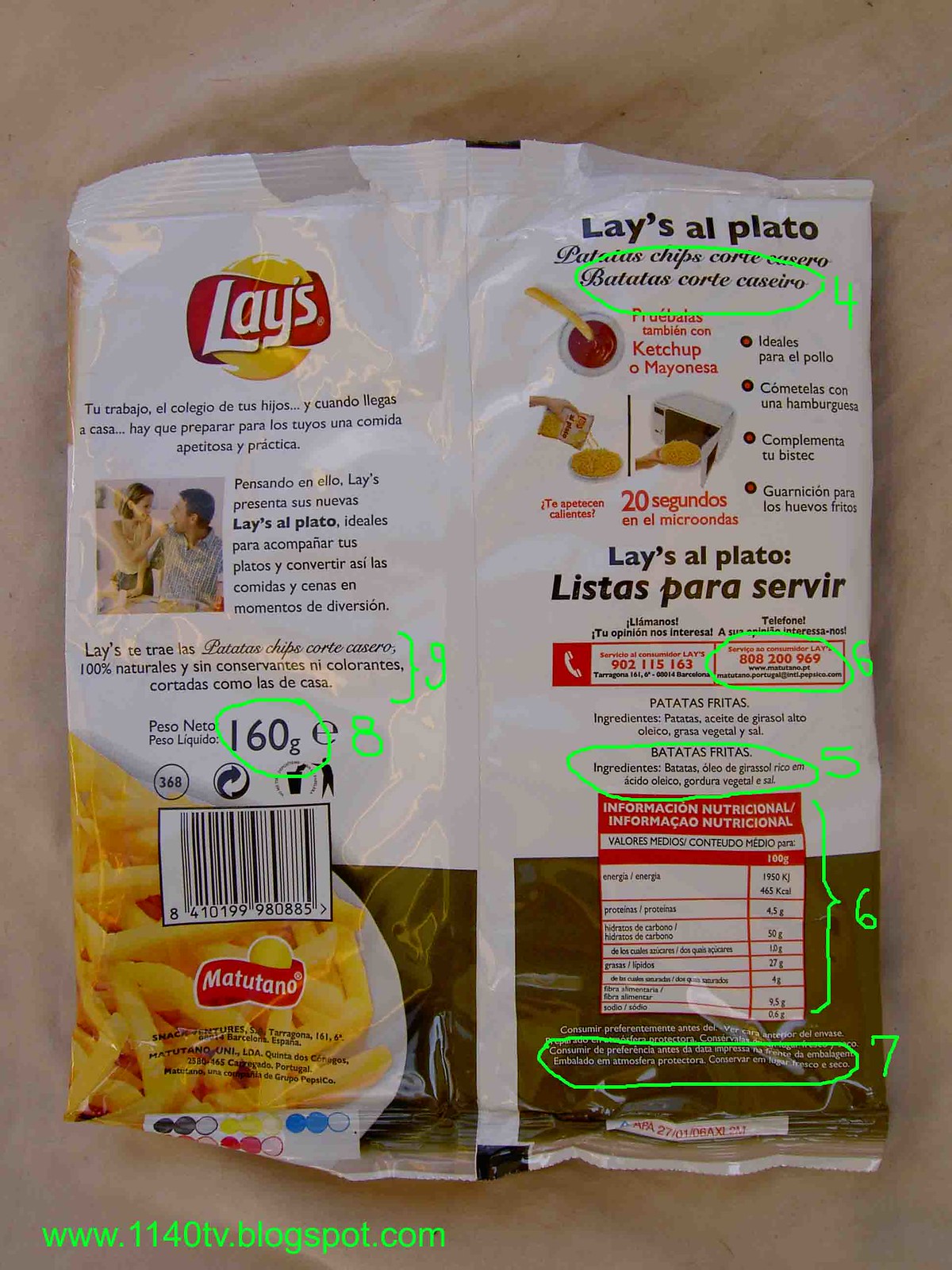The image features a Lay's potato chip bag laid flat with the back side facing up. The packaging is printed in a different language, yet the recognizable Lay's logo is prominently displayed. A white dish with food is pictured on the back of the bag. Various sections of the bag are circled in neon green and labeled with numbers ranging from four to nine. These include the following highlighted elements: 

- The weight indicated as 160 grams.
- A phone number.
- An inscription at the top of the bag, although it is indecipherable.
- The fine print near the middle of the bag, labeled as seven.
- The nutrition label, which is marked as six, featuring red font with black lettering on a white background.

Additionally, the website "www.1140tv.blogspot.com" is also visible.